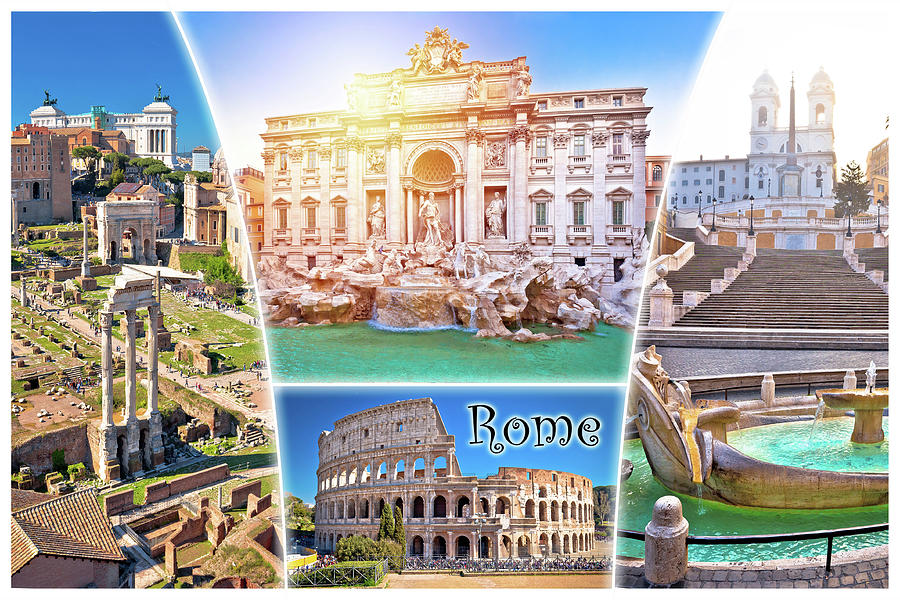The collage features four vibrant and lively photographs, arranged in a rectangular landscape format with the top and bottom sides being twice as long as the left and right sides. On the far left, the image showcases ancient Roman ruins with multiple columns and foundations, juxtaposed against a backdrop of modern buildings under a blue sky. The far-right image captures a man-made water fountain with clear blue water, leading up to the iconic Spanish Steps, and culminating at a double-towered church above. Centered at the top is a grand palace-like structure adorned with statues and fronted by an expansive man-made waterfall fountain, evocative of the Trevi Fountain. Meanwhile, the bottom center image prominently displays the Colosseum under a bright blue sky, accompanied by large black text reading "Rome," highlighting the iconic nature of this historical site. Together, these images encapsulate the architectural grandeur and tourist allure of Rome, blending both ancient and modern elements in a captivating and colorful montage.